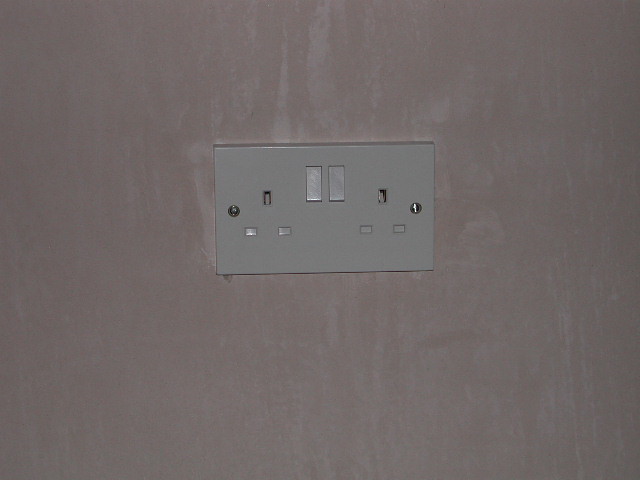This detailed image showcases a white, 2-gang, 13A double switched power electric socket installed on a piece of white drywall. The electrical socket features two three-prong plugs, each situated on opposite sides of the device. The center of the socket is characterized by two rectangular switches. There are also silver screws visible—one on each side of the socket, securing it firmly to the wall. The image predominantly contains colors such as white, off-white, and silver, and the socket's plastic plate is positioned centrally in the image. The setting appears to be indoors, likely inside someone's house, with the entire scene composed against a solid white background. There are no identifying texts or additional objects visible in the photograph.